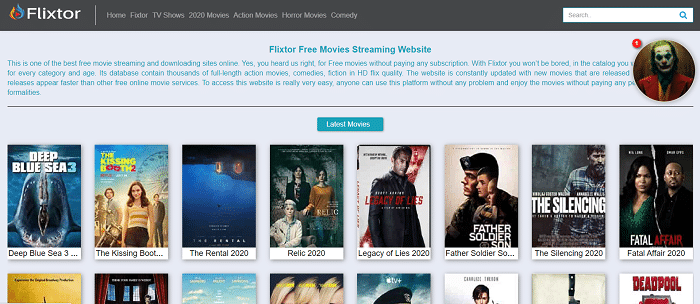**Caption:**

A screenshot of the Flickster website showcases its interface and offerings. At the top left, the site's name "Flickster" is prominently displayed with a small fire icon next to it, symbolizing hot or trending content. The navigation bar includes options such as "Home," "TV Shows," "2,000+ Movies," "Action Movies," "Horror Movies," and "Comedy." Flickster is branded as a premier free movie streaming and downloading site, emphasizing that users can access a vast array of movies without any subscription fees. The site boasts a comprehensive catalog that caters to all categories and age groups, featuring thousands of full-length action movies, comedies, and fictions, all in high-definition (HD) quality. Flickster's database is regularly updated, ensuring that new releases are available faster than on competing free movie services. The interface is designed to be user-friendly, making it accessible to anyone without complications. Displayed on the screen are some of the latest movie titles available, including "Blue Sea 3," "The Kissing Booth," "The Rent-A-Phone (2020)," "Alexia Lies (2020)," "Father Soldier Son," "The Silencing," and "Fatal Affair."